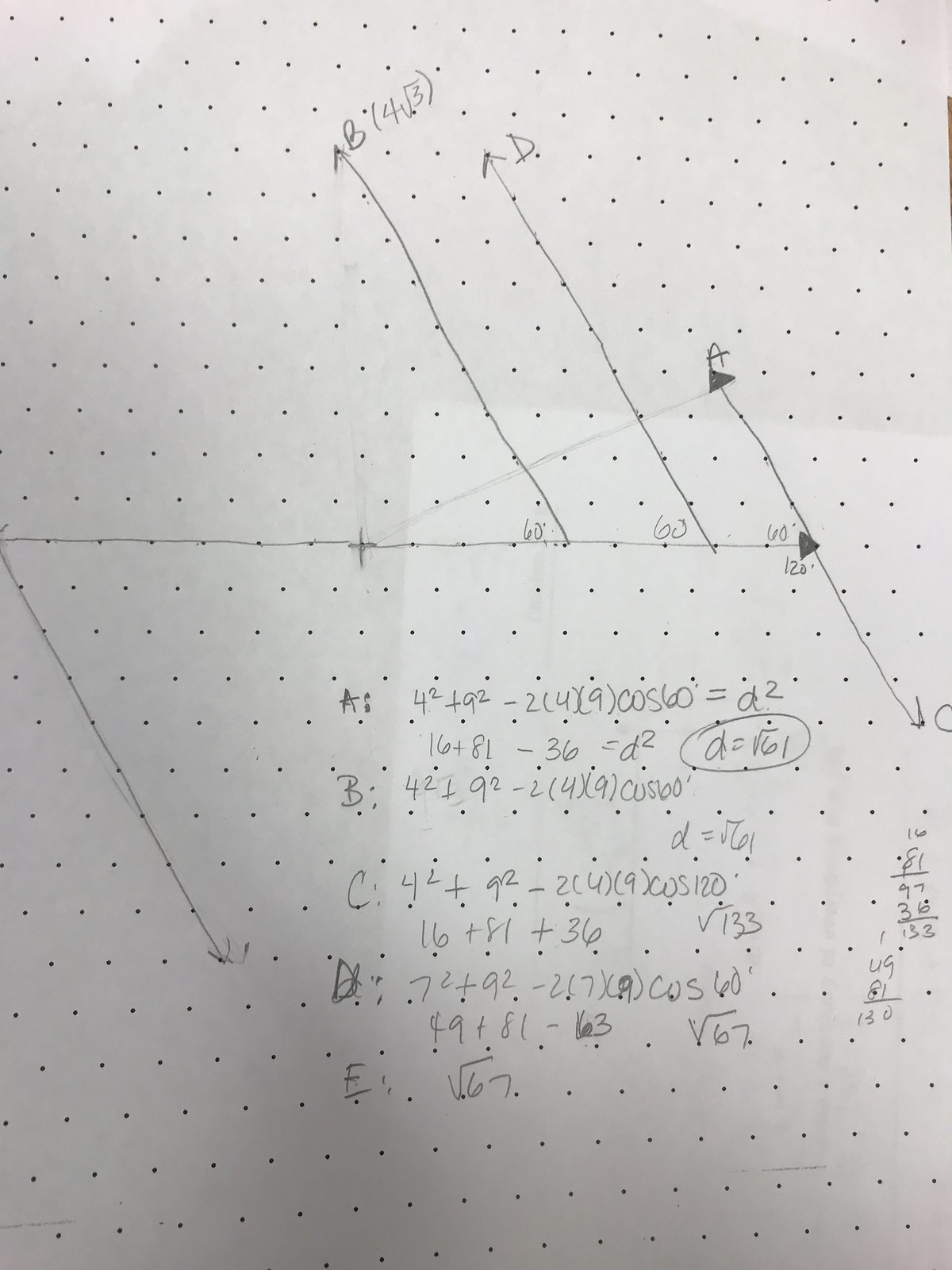This image features a detailed handwritten sketch and associated calculations, likely related to a geometry or physics problem, meticulously drawn on graph paper with a dotted grid. The central focus is a diagram comprising vectors or lines, meticulously labeled with the letters A, B, C, D, and a specific point marked RB 14.5. These vectors depict various directions and magnitudes within a coordinate system or vector space, intricately connected at specified angles of 60° and 120°. 

The hand-drawn nature of the lines and angles suggests this is either a conceptual sketch or the preliminary stages of problem-solving. Beneath the diagram are extensive mathematical calculations employing the law of cosines to determine the distances between points. Each calculation is carefully labeled pertaining to different points or vectors from A to E, involving complex square roots and cosine functions. This detailed depiction not only highlights the analytical approach but also the methodical process in solving a sophisticated geometric or physical problem.